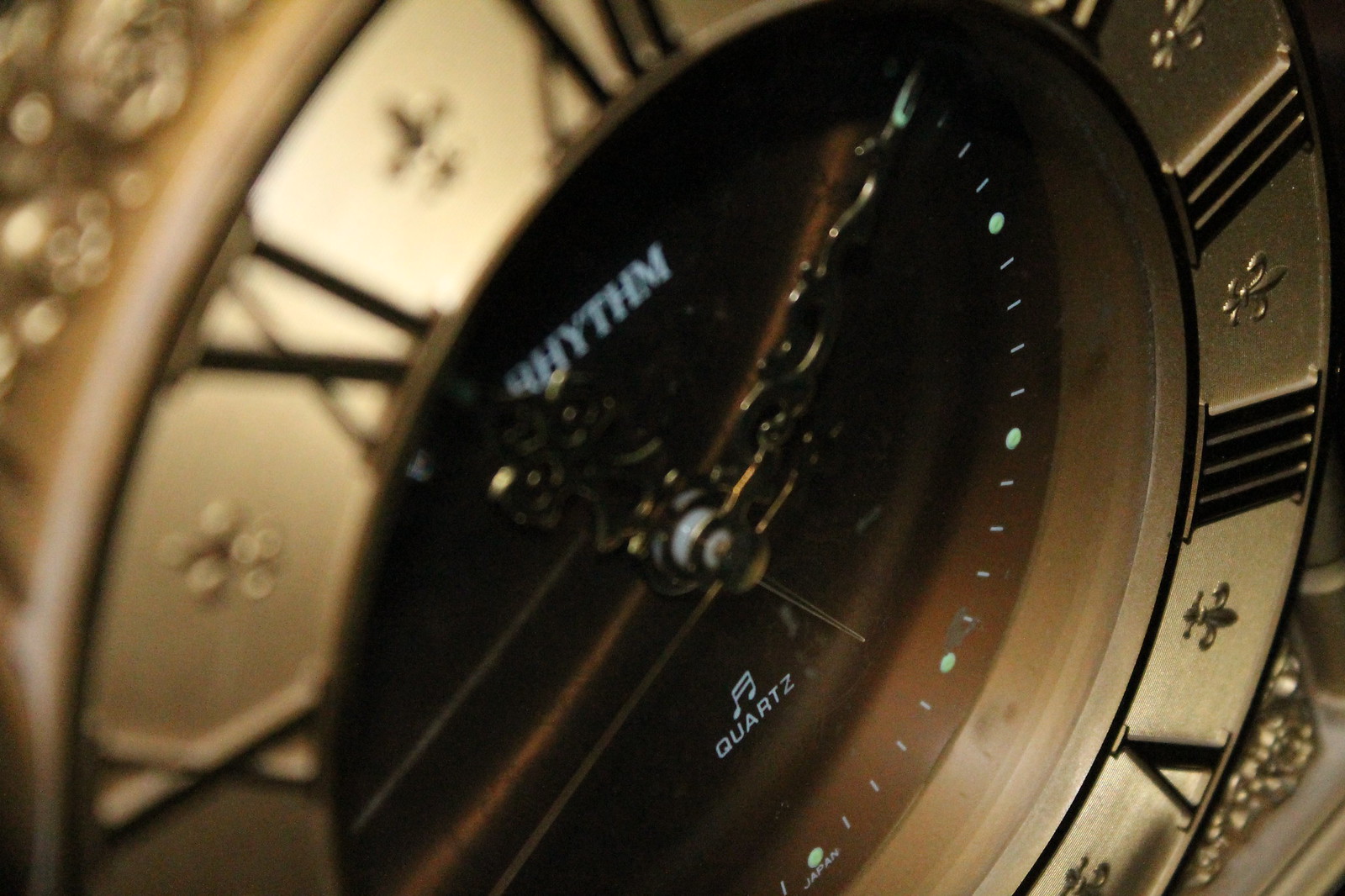A detailed close-up image captures the face of a watch, presenting it at a left-tilted angle. The closest part of the watch face is positioned on the left side of the frame, with the perspective extending diagonally to the right, creating a dynamic composition. The upper portion of the watch, nearest to the camera, appears blurred, gradually coming into sharp focus as the view shifts away from this point. The watch boasts a sophisticated black face, contrasting elegantly with its encircling gold-colored bezel. Inscribed on the watch face is the word "Rhythm," prominently displayed, while the bottom segment features the text "Quartz" accompanied by a delicate musical note symbol, reflecting the watch's precise and artistic design.